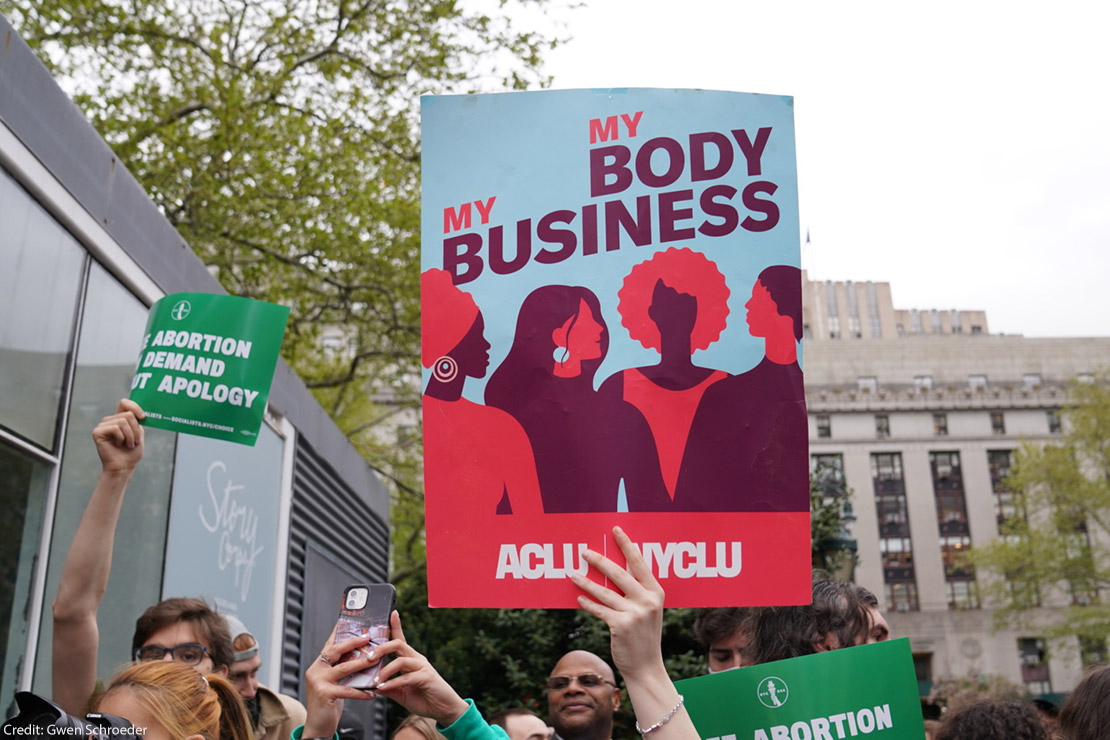This photograph captures a detailed scene of an outdoor pro-abortion protest. Central to the image is a woman's hand holding up a sign that reads "My Body My Business," attributed to the ACLU and NYCLU. The poster features a blue background with red and purple figures, possibly representing women or individuals identifying as women, depicted in a corporate cartoon style, standing next to a black building. To the left, another woman is seen holding up her phone with both hands, while a man beside her holds a green sign with partially readable white lettering stating "Abortion Demand Apology." The background reveals the tops of protesters' heads, a large government-like building with classical architecture, and green tree tops, adding depth to the bustling and fervent protest atmosphere.